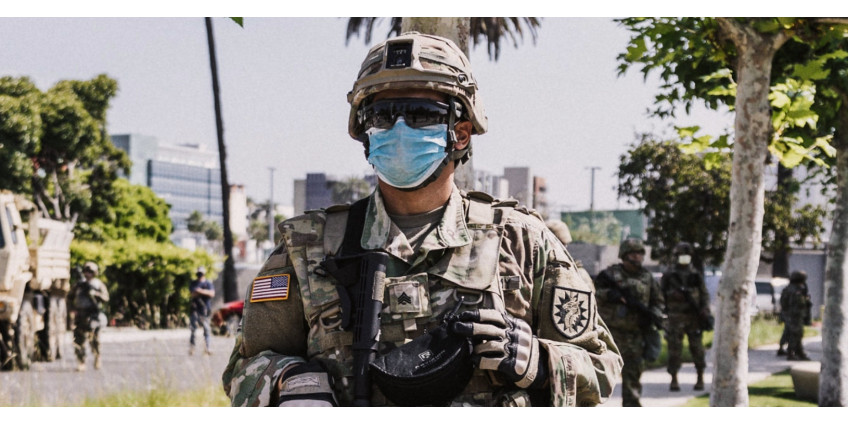The photograph features a U.S. soldier positioned centrally, clad in full combat gear, including a khaki-colored uniform, helmet with an attached camera, black wraparound protective sunglasses, a blue medical face mask, and gloves. On his left shoulder is an American flag patch, and on his right shoulder, a different insignia is visible. He is surrounded by various equipment, the precise nature of which is unclear. Behind him, the background is blurred but reveals several other soldiers similarly attired in light-colored camouflage, along with what appears to be a beige-armored vehicle, possibly reminiscent of a Bradley. The setting includes dense trees, some resembling palm trees, and indistinct office buildings, indicating a complex environment, though the exact location remains unspecified.